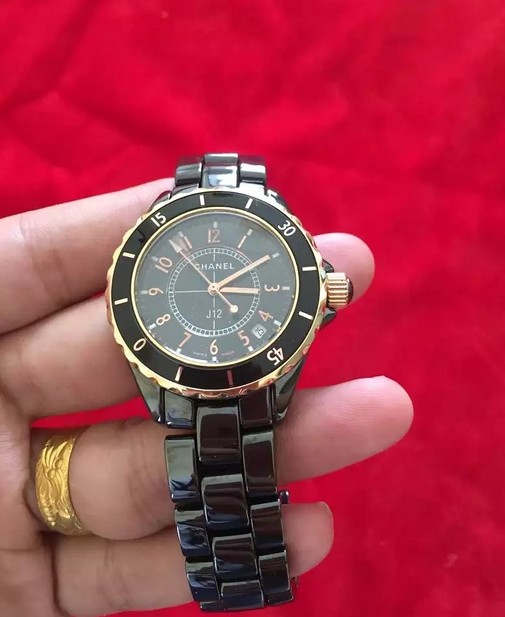This close-up photograph captures a black Chanel wristwatch with an attention to intricate details. The watch, positioned centrally, is draped across the index and middle fingers of a hand, with the band wrapping around the rest of the fingers. The hand, shown palm up, has a gold embossed ring on the ring finger. The background is a vivid red, contrasting sharply with the glossy black of the watch. The watch's face is predominantly black, featuring gold hands and red numerals at intervals along the dial, particularly highlighting the external numbers: 0, 15, 30, and 45 in gold. The watch face also displays the brand name "Chanel" and the model designation "J12." The wind-up knob, located on the right side, is distinguished by its ridged texture and gold accent. It's almost ten minutes past three, as indicated by the hands on the face.